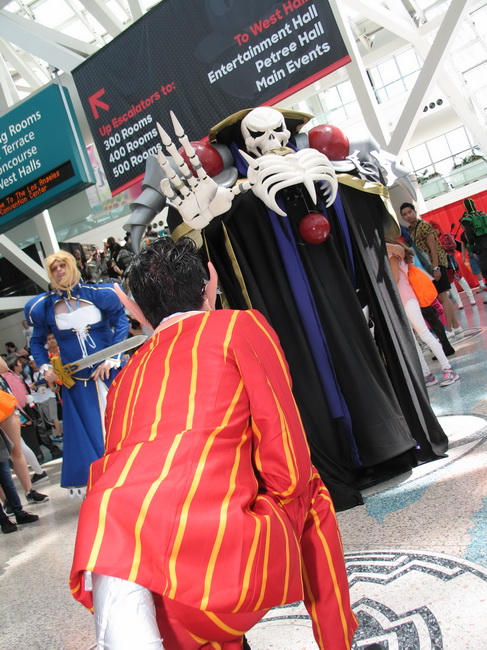In a bustling convention hall, reminiscent of events like Comic-Con or Dragon-Con, a young man in an elaborate red suit with yellow stripes and long elf ears kneels down reverently. His attire, with intricate patterns and possibly a tail, adds to the striking ensemble. He bows before an imposing figure clad in a detailed Grim Reaper costume, complete with a skull mask, oversized skeletal hands, a ribcage, and a black and purple cape with brown triangular hair tufts. This menacing character is recognizable from the Overlord anime. To the right, another cosplayer stands, wielding an oversized sword and donning a blue dress with a blonde wig, perhaps portraying a character from Japanese manga. The scene is set against a backdrop of signs indicating directions to various rooms and halls, suggesting the extensive layout of this dedicated anime convention. A diverse crowd, also in vibrant costumes, mills about, captivated by the display, highlighting the communal spirit and shared enthusiasm for cosplay.